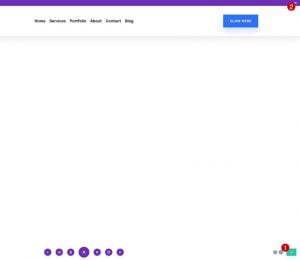The image depicts a blurry screenshot of a website interface, making the text difficult to read due to its tiny size. Starting from the top right, there's a prominent purple header bar featuring a red symbol or icon at its end. Below the header is a rectangular section containing five different menu options. Among these menu choices, the items "Blog" and "About" are faintly readable. 

In the lower section of the image, there's a notable blue key button. Underneath the button, six small purple circles are arranged on the lower left side. Each circle contains a white symbol that is indecipherable due to the blurriness. The entire background of the website is white, further accentuated by the minuscule text throughout.